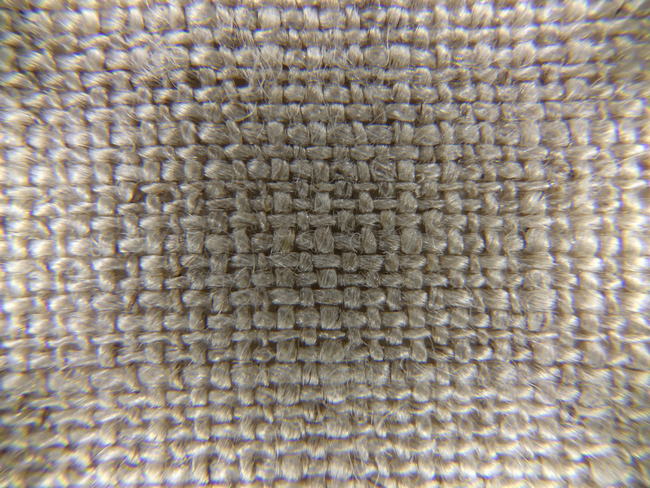This extreme close-up image showcases the intricately woven texture of a thick, tightly woven textile, possibly resembling fabric, gauze, or a rug. The majority of the material is a light sand brown or taupe color, characterized by a well-defined weave pattern. The center of the image is noticeably darker, creating a focal point that might result from shadowing or the presence of a camera overhead, while the edges appear blurry, enhancing the central focus. There's a notable difference in coloration and texture between the center and the corners, suggesting either soiling or variation in the light reflection. The image lacks any form of border, labeling, or other elements, emphasizing the detailed woven fibers, which appear either densely knitted, resembling wool or rope, or synthetic, with a somewhat rough texture. The absence of any patterning indicates a basic, yet intricate weave, contributing to the overall texture-centric presentation.